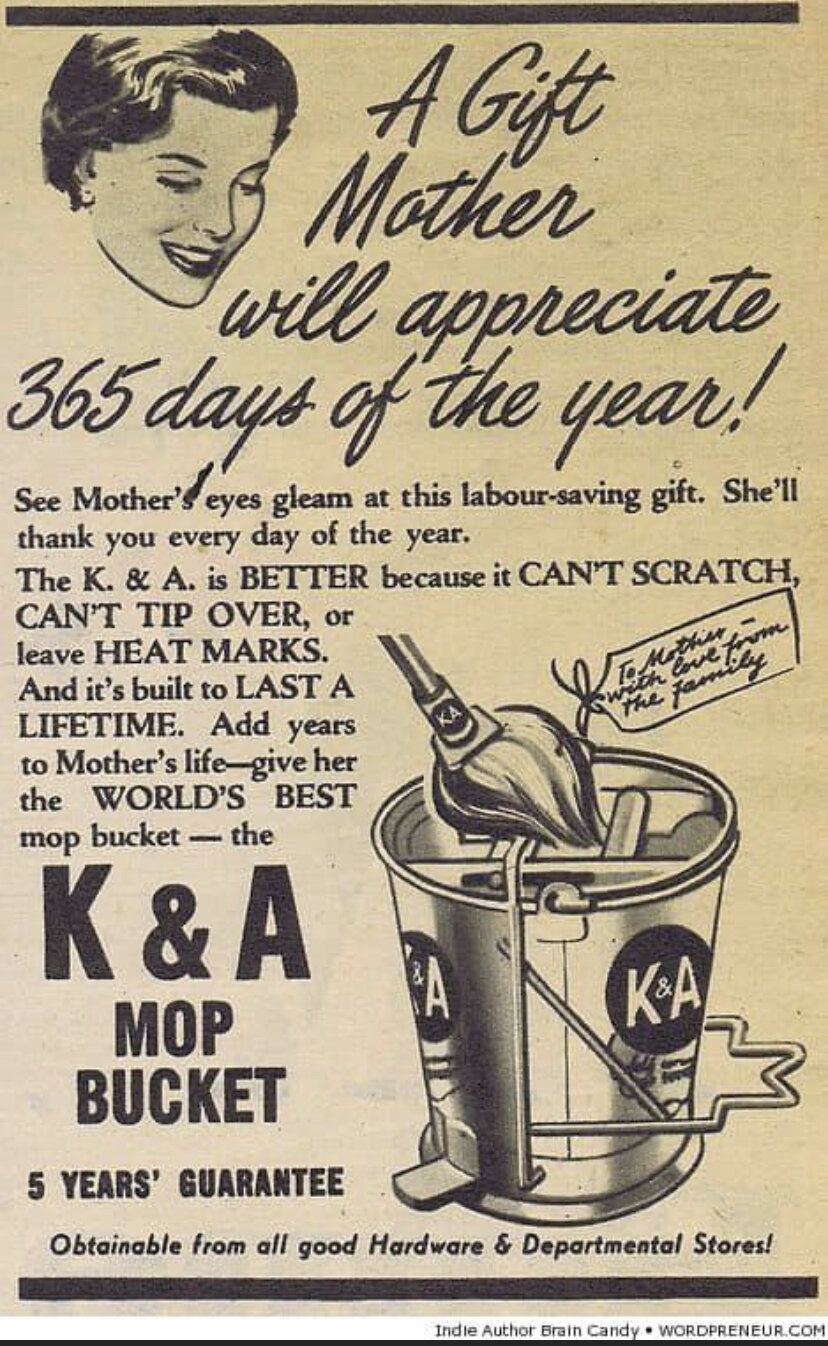The image presents a vintage newspaper advertisement on yellowed paper with black ink, bordered by thick black bands at the top and bottom. In the upper left corner, there's an illustration of a woman with short, dark brown hair, smiling and looking downward. The prominent headline in italicized script reads, "A gift Mother will appreciate 365 days of the year!" Accompanied by the tagline, "See mother's eyes gleam at this labor-saving gift. She'll thank you every day of the year!" 

The centerpiece of the ad showcases the K&A mop bucket, touted as being superior because it "can't scratch, can't tip over, or leave heat marks," and is "built to last a lifetime." The ad promises to "Add years to Mother's life" by giving her "the world's best mop bucket." The bucket itself is metal with a step-operated squeezer, and a mop is illustrated placed inside it. A tag attached to the bucket reads, "To mother with love from the family." Bold text at the bottom declares, "K&A mop bucket," and emphasizes a "Five-year guarantee." The product is advertised as "obtainable from all good hardware and department stores," and at the base of the ad, there is a note mentioning, "Indie author, brain candy, worldpreneur.com."